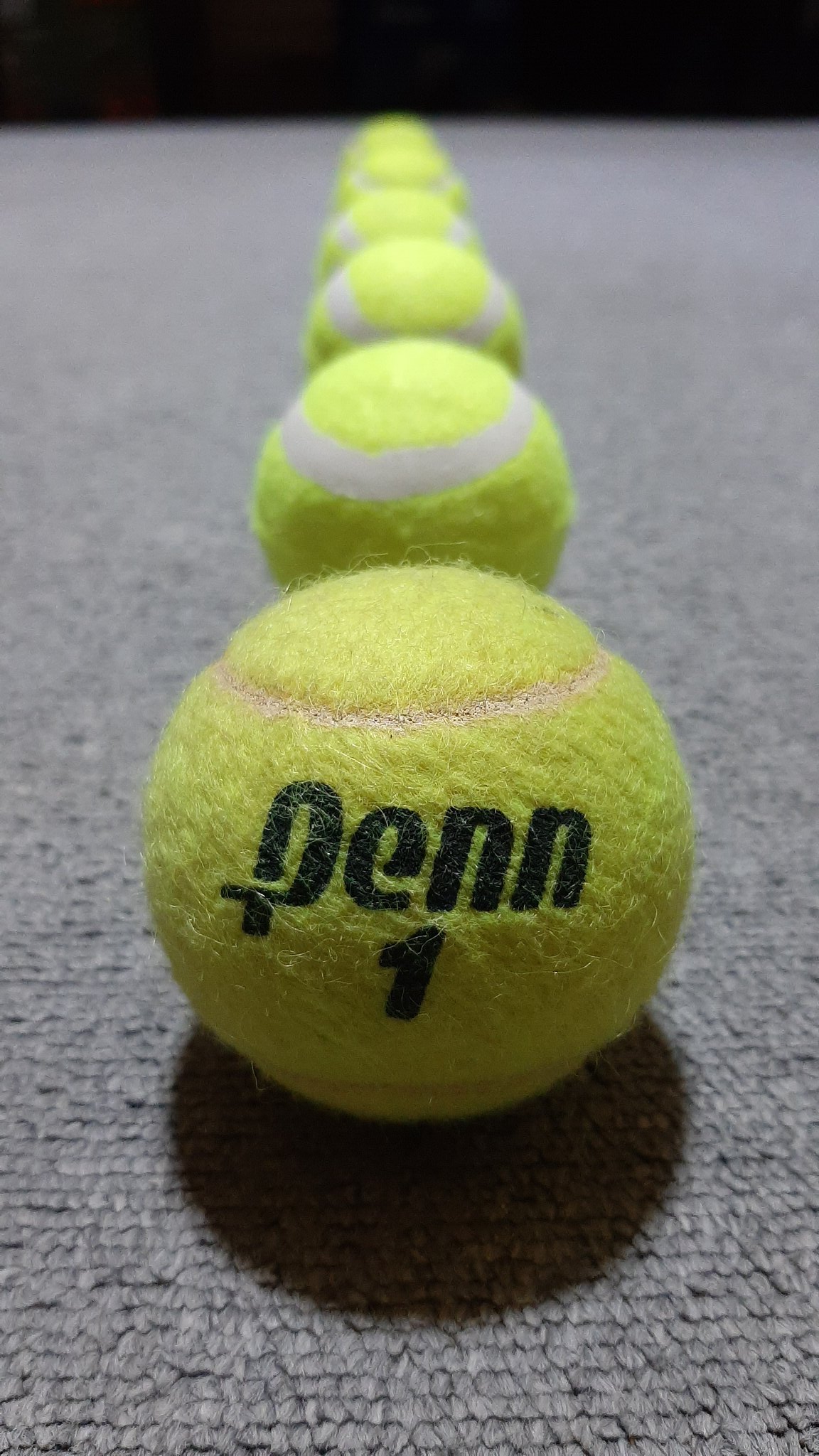The photograph features a long, vertical composition showcasing a row of tennis balls meticulously arranged in a straight line on a gray carpet. The balls themselves are a vivid yellow-green color with white stripes. The focal point is the nearest ball, which is sharply in focus, revealing the black text "P-E-N-N 1" on its surface. As the eye moves toward the background, the remaining five or six tennis balls gradually blur into obscurity. A shadow cast by the light source enhances the texture of the foremost ball and the carpet beneath. The background at the top edge of the image fades into a stark black line, contrasting sharply with the textured gray carpet below.